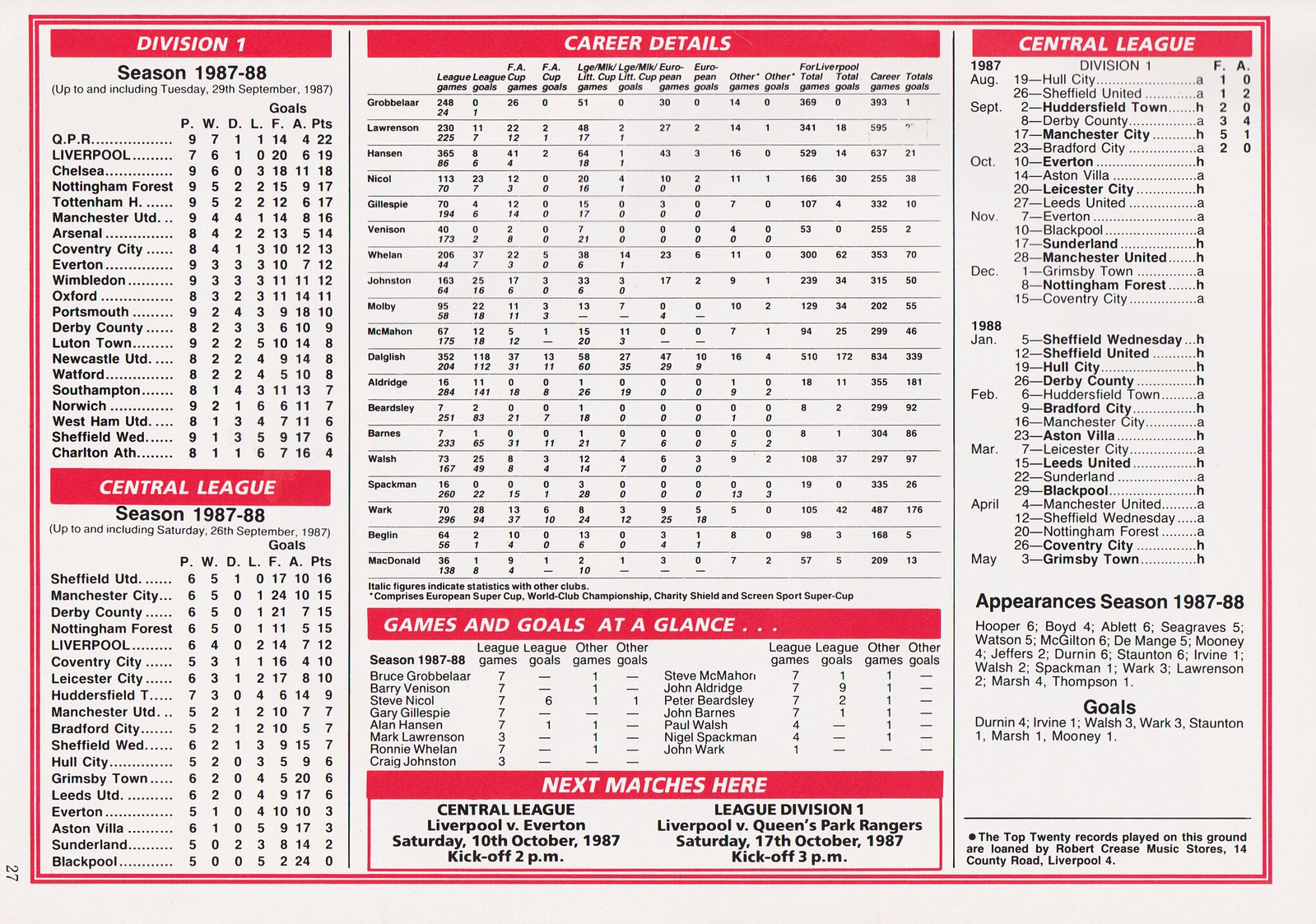The image is an old white card with red trim from the 1987-1988 English football season, featuring a detailed chart divided into three columns. The left and right columns are narrower, and the middle column is wider. Each section has a red banner with white text highlighting key information. The left column starts with "Division One" and "Season 1987-1988" in black, listing various soccer teams, including Sheffield United and Manchester City. Below, "Central League" is highlighted in a red banner, followed by team names and player stats. In the center column, a red banner titled "Career Details" lists various players and their statistics. This is followed by another red banner reading "Games and Goals at a Glance," summarizing player performance. At the bottom, another red banner reads "Next Matches Here," detailing upcoming fixtures: Liverpool vs. Everton on October 10th, 1987 at 2 PM, and Liverpool vs. Queens Park Rangers on October 17th, 1987 at 3 PM. The right column begins with "Central League" in a red banner, followed by more team statistics under "1987 Division One." The card efficiently summarizes how teams and players are performing in this particular season.